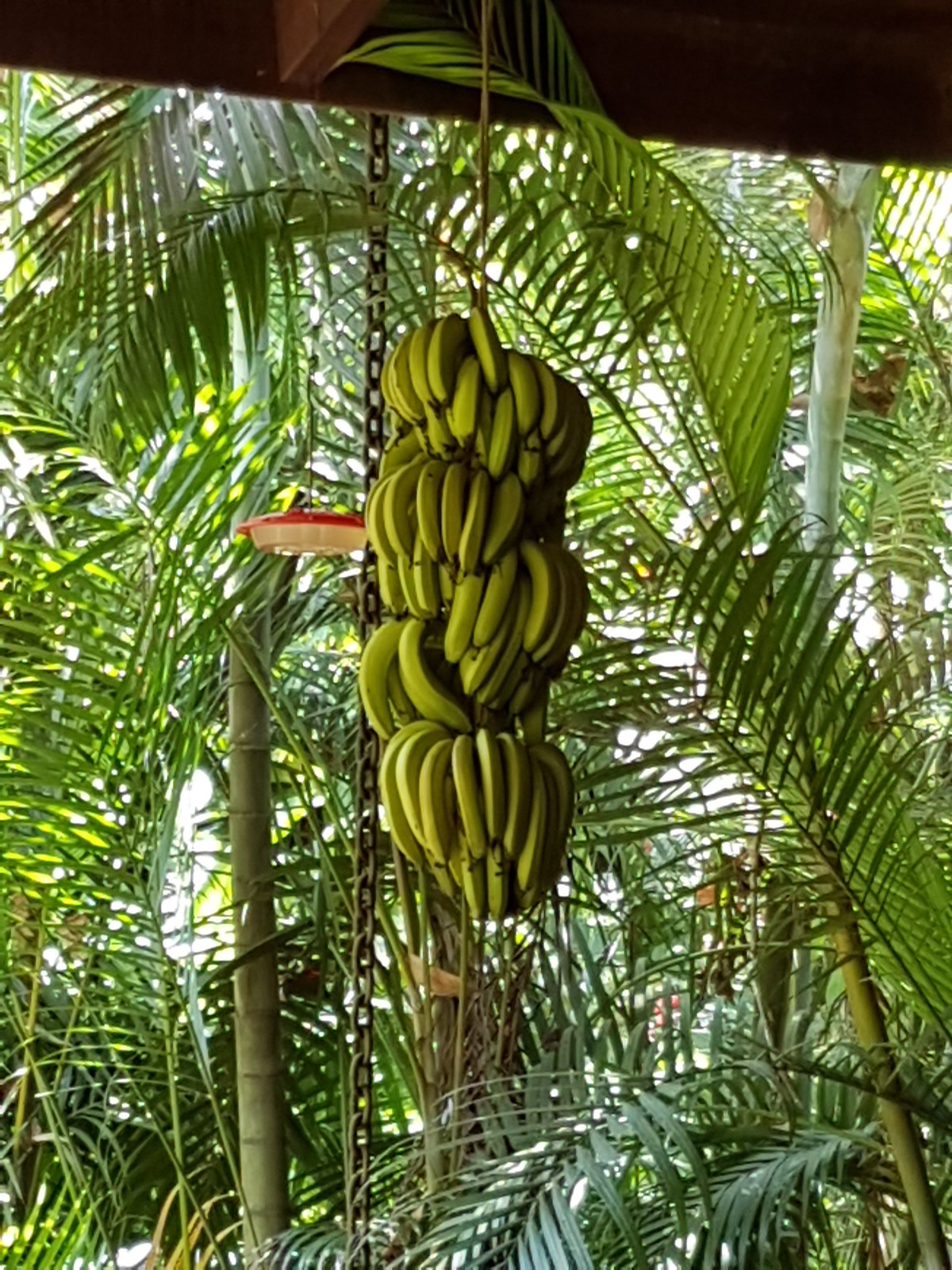The image depicts a large bunch of bananas hanging from a cable tied to a brown wooden awning or roof. The bananas, clearly freshly cut from a tree, are predominantly green with a slight yellow hue and some brown tips, indicating they are not yet fully ripe. Surrounding the bananas is a lush, jungle-like setting with numerous palm leaves and slim tree stems extending upwards from the ground. A noticeable gray metal chain runs from the roof to the ground alongside the bananas. The bunches, organized into about five rows, contain numerous bananas, possibly totaling up to a hundred or more. This scene conveys a tropical, outdoor ambiance, reminiscent of a patio or garden area.